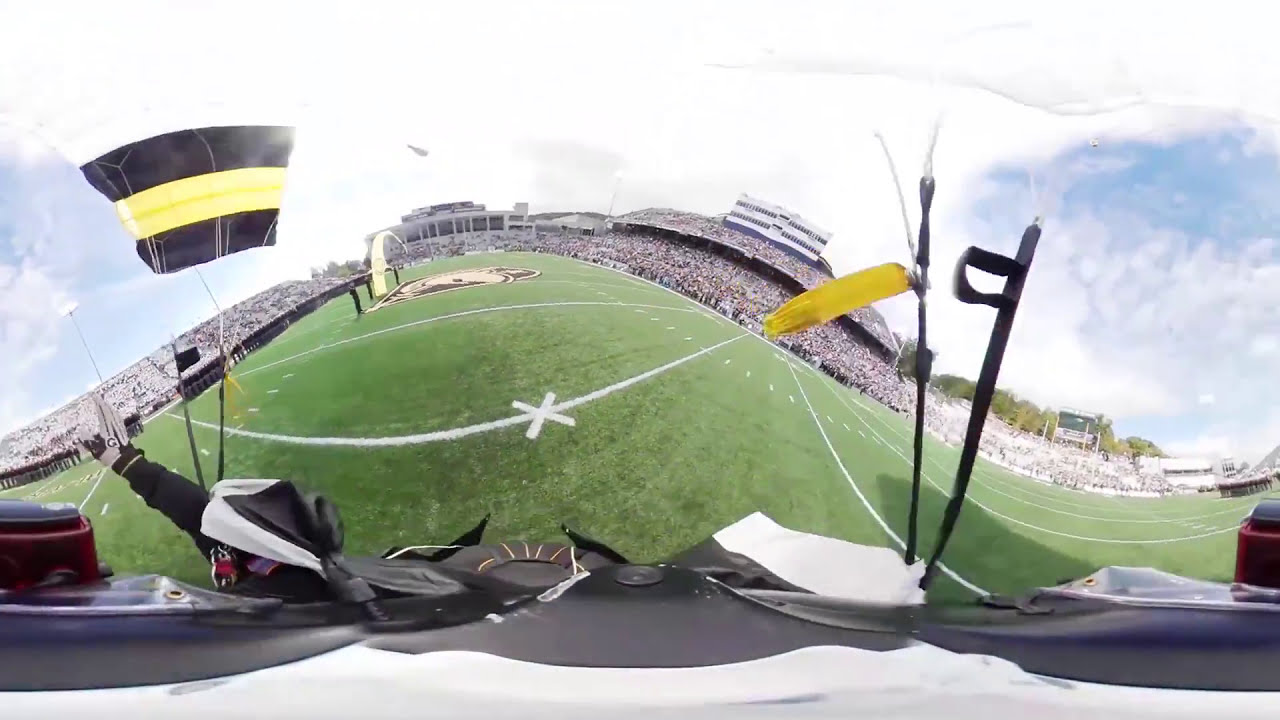A panoramic image captures a football stadium on a sunny day with a few clouds in the blue sky. A man is parachuting onto the lush green field, his arm reaching up, possibly waving to the crowd. Black, yellow, and white cords connect him to the parachute, matching the colors seen on flags around the stadium and on parts of the field. The parachute itself is partially visible on the left side of the image, though it's cut off by the panorama. You can see the man's chest and one hand, with ropes stretching upwards, making it clear he's landing at the center of the field, marked by a white X. The field also features a team logo near the drop zone. Across the field, there are two levels of packed stands filled with onlookers, their faces eager as they watch the descent. A large building with pillars stands prominently in the background, adding to the grandiosity of the scene.